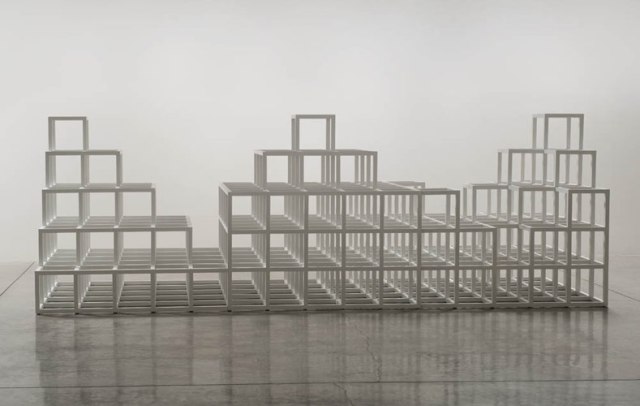This photograph captures a modern, abstract art installation composed of numerous white, wired-frame cubes stacked together on a reflective white marble gray surface. The background is a clean, minimalist white wall that enhances the starkness and modernity of the piece. The arrangement of these transparent cubes conveys a three-dimensional grid, resembling a miniature cityscape with a sense of both regularity and unevenness. 

From left to right, the cubes are stacked in varying heights, specifically following this sequence: 5, 4, 3, 2, 1, 3, 4, 5, 4, 3, 3, 2, 3, 4, 5. They are aligned in a way that spans at least 15 cubes wide along the bottom and extends six cubes deep, with the right side of the structure angled to display the depth of the arrangement. 

The lighting in the room creates a dim ambiance, causing the white cubes to exhibit different gray gradations and shadows. The most pronounced shadows are cast by the bottom layer of the cubes and their reflections on the polished marble-like floor, adding to the visual complexity and depth of the sculpture.